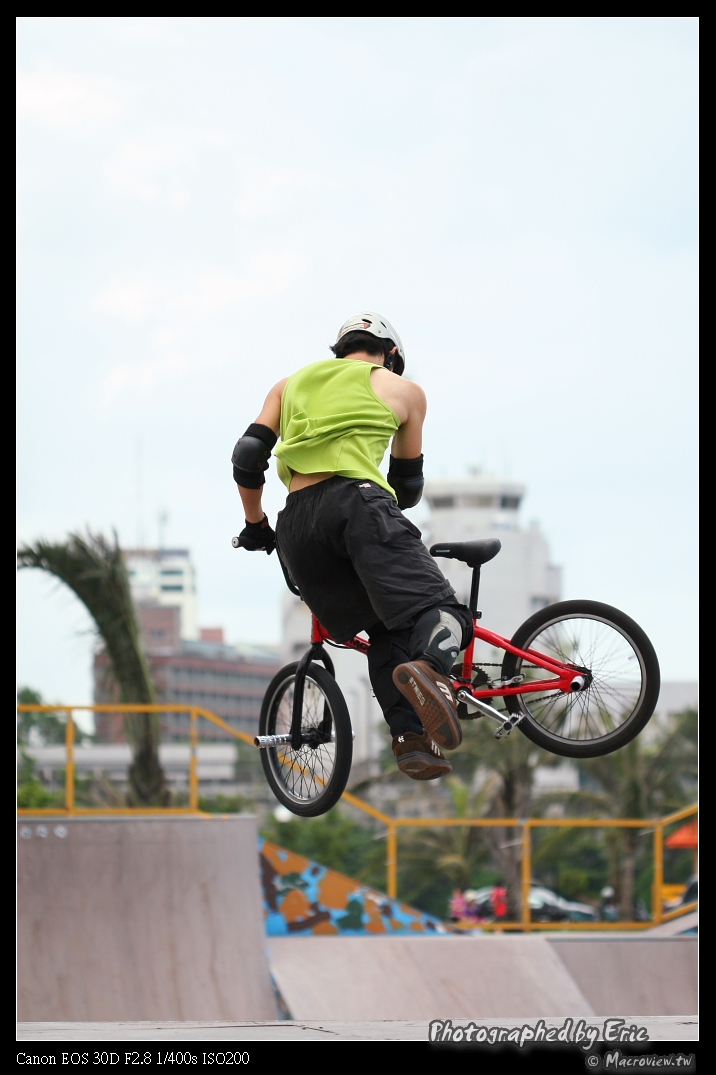In this dynamic outdoor action shot, a BMX rider, clad in a lime green tank top and black shorts, soars through the air mid-stunt. He sports comprehensive protective gear, including black elbow pads, sleek black gloves, and full lower leg pads, complemented by brown tennis shoes. His eyes are fixed downwards towards his red BMX bike, which is nearly perpendicular to his body, with his hands gripping the handlebars and his feet off the pedals. His bike features black tires and pegs protruding from both wheel hubs, ideal for performing various tricks. The background reveals the vibrant setting of a skate or bike park, marked by ramps, yellow railings, and lush palm trees. Further back stand two large buildings; one is notably octagonal at the top resembling an airport control tower, while the other appears like a brick parking garage with expansive open sections. The clear sky creates a picturesque horizon a third of the way up the frame. A watermark "Photographed by Eric at Macroview.tw" features prominently, and technical details in the bottom left corner indicate the photo was taken with a Canon EOS 30D F2.8 1/400 ISO 200.